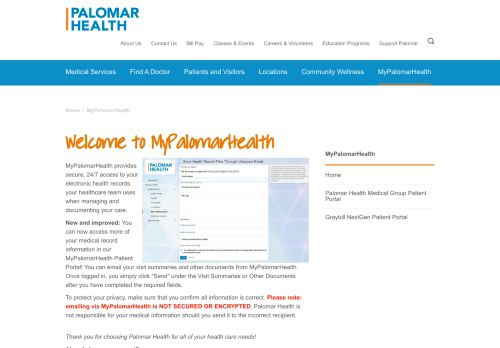This screenshot is from the MyPalomarHealth section of the Palomar Health website. It welcomes users and informs them that MyPalomarHealth offers secure, 24/7 access to their electronic health records. This feature allows users to manage and view their health information online conveniently. The website emphasizes the importance of using a secure computer when accessing MyPalomarHealth, as the information is not encrypted. Additionally, the page provides links to other sections of the site, including medical services, finding a doctor, and patient and visitor information.

At the top of the website, there's a blue bar with navigation tabs that include Medical Services, Find a Doctor, Patients and Visitors, Locations, Community Wellness, and MyPalomarHealth. Above this blue bar, further navigation options are listed, such as About Us, Contact Us, Bill Pay, Events, Careers and Volunteers, Education Programs, and possibly a festival link. The MyPalomarHealth section is highlighted, showing some introductory text that provides information on how to log in and use the services.